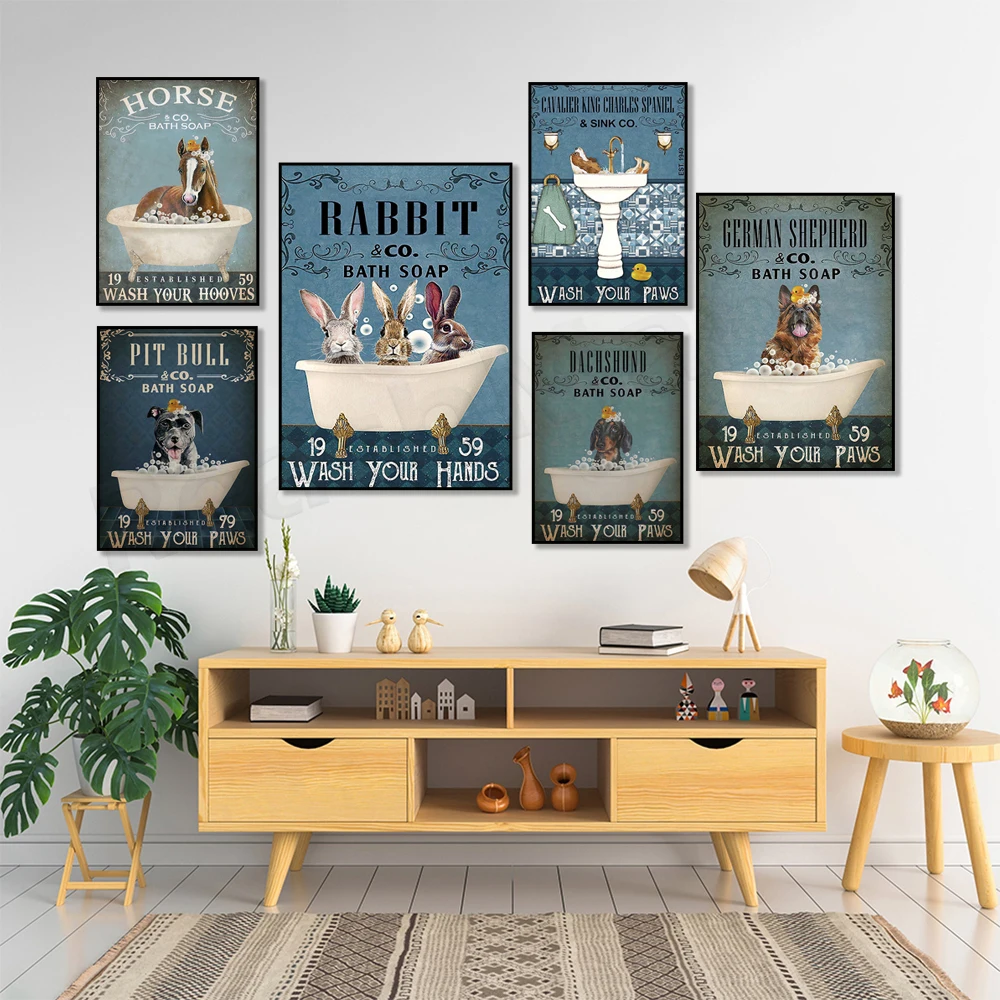The image depicts a stylized, computer-generated living room with a white-tiled floor adorned with a gray, woven rug. Central to the setting is a white wall decorated with a series of 6 framed posters, each featuring whimsical illustrations of various animals in vintage-style bathtubs or sinks. The posters, arranged in a gallery-like fashion, advertise fictional bath soaps with playful slogans. From left to right, the sequence includes a horse with the caption "Horse and Company Bath Soap: Wash Your Hooves," followed by a pitbull stating "Pitbull and Company Bath Soap: Wash Your Paws." A larger poster of a rabbit reads "Rabbit and Company Bath Soap: Wash Your Hands," flanked by images of a dachshund and a German shepherd in bath settings, all maintaining a cohesive blue-hued theme.

Below the posters is a TV console with two shelves and pull-out storage compartments, displaying an array of decorative items such as books, a lamp, miniature bird figurines, a small succulent, and some flowers. To the left of the console sits a small table holding a lush monstera plant, while to the right, a similar table supports a bowl containing a few fish. The overall atmosphere is commercial yet cozy, blending modern and vintage elements in a harmoniously stylized space.